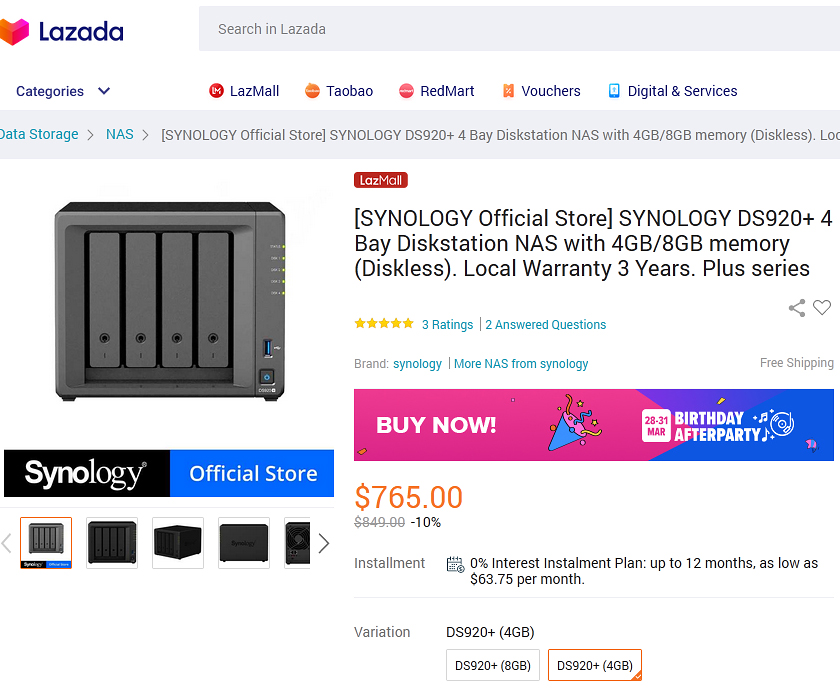This screenshot captures a website with a white background. In the upper left corner, there is a logo comprising a red "V" followed by the word "Lazada" in blue font. Adjacent to the logo on the right is a gray search field containing the placeholder text "search in Lazada" in darker gray font. Below this, there is a navigation bar starting with a drop-down menu labeled "categories," followed by clickable links for "Lazamal," "Taobao," "Redmart," "vouchers," "digital," and "services."

Further down, a gray rectangular section features the text "data storage" in blue font, accompanied by a forward arrow, leading to "NAS," followed by another forward arrow. This sequence directs to the "Synology official store" in black font, specifically highlighting the "Synology DS 920+ 4 bay disk station NAS with 4GB/8GB memory (diskless)." Beneath this, an indicator in a red square says "Lazamal."

To the left of this description, there is a photo of the product, which appears as a gray box with buttons on it. To its right, in black font, the text reiterates the "Synology official store" and the product details: "Synology DS 920+ 4 bay disk station."